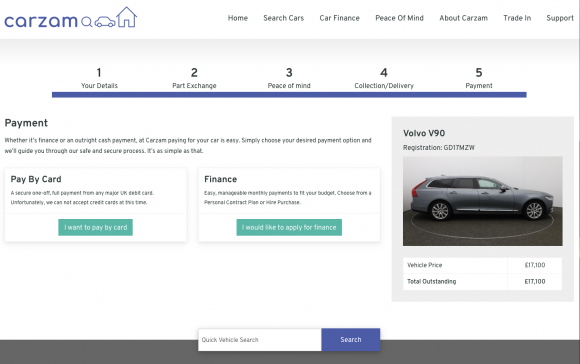The image features a predominantly white background with various colored text and graphics organized across different sections. 

At the top, centered, is the text "Car Zam" in blue. Adjacent to it is a blue magnifying glass icon, followed by the outlines of a car and a house. 

On the right hand side, there is a list of navigation options in black text: "Home," "Search Cars," "Car Finance," "Peace of Mind," "About Car Zam," and "Trade and Support."

A gray section beneath these headers includes a sequence numbered one through five in black. Below each number are steps labeled: "Your Details," "Part Exchange," "Peace of Mind," "Collection/Delivery," and "Payment." This section is demarcated by a thicker blue line.

Continuing on the white background, black text on the left reads "Payment." This section explains that whether paying via finance or outright cash, Car Zam provides an easy, safe, and secure method. It reassures users with, "Paying for your car is easy. Simply choose your desired payment option, and we'll guide you through our safe and secure process. It's as simple as that."

Below this, two payment options are detailed:
1. **Pay by Card**: Described as a secure, one-off full payment from any major UK debit card, though it notes the inability to accept debit cards at this time. This option is emphasized with a teal green button labeled in white text, "I want to pay by card."
2. **Finance**: Offering manageable monthly payments suited to the user's budget, with choices between a personal contract plan or hire purchase agreement. This option also has a teal green button labeled in white text, "I'd like to file for finance."

The focus then shifts to a specific car, a gray Volvo V90, priced at £17,100.

At the bottom center, there's a quick vehicle search guide, accented by a blue button with white text that says "Search." Below this is a darker green bar spanning across the width of the section.

The design is thoughtfully laid out to guide the user through a comprehensive and user-friendly experience, simplifying the car purchasing process at Car Zam.